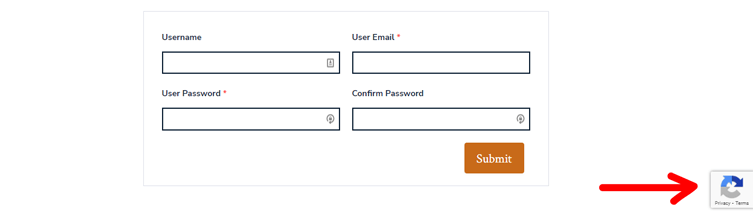This image is a detailed screenshot of a sign-in form interface with various input fields and annotations. The sign-in form consists of a rectangular box with a thin, faint gray border. Inside this box, there are four labeled text fields organized in a grid pattern:

1. **Upper Left:** The first field is labeled "Username" and features a rectangular input box for typing in the username.
2. **Upper Right:** Adjacent to the "Username" field is the "User Email" field, which includes a red asterisk indicating that entering an email is mandatory.
3. **Lower Left:** Below the "Username" field is the "User Password" field, also marked with a red asterisk to signify that it is required.
4. **Lower Right:** Next to the "User Password" field is the "Confirm Password" field.

Beneath these fields, on the lower right, there is a button with rounded corners in an orangeish-brown color that reads "Submit" in white font.

Additionally, a red arrow points toward a "Privacy Terms" box located along the bottom of the image. This box contains an icon of three arrows forming a circle, colored in gray, light blue, and dark blue, drawing attention to the privacy terms. The purpose of the red arrow annotation is unclear, but it suggests the importance of reviewing the privacy terms in the context of this form.

Overall, this screenshot appears to depict a sign-in process requiring users to input a username, email, password, and password confirmation, with an emphasis on understanding privacy terms.